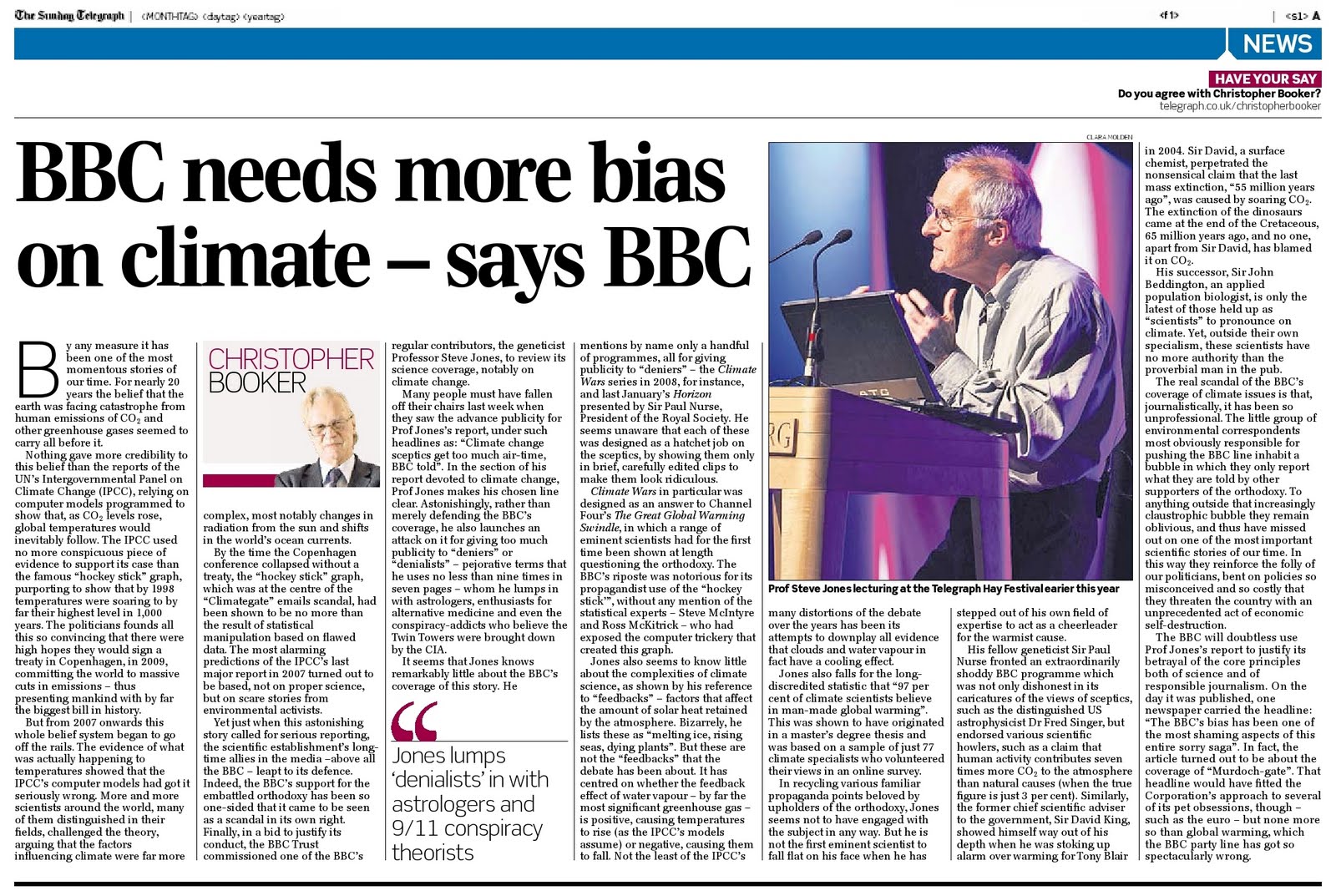The image displayed on the website features a newspaper clipping with an article titled "BBC Needs More Bias on Climate, Says BBC" in large, bold letters. The article is authored by Christopher Booker. The top of the clipping shows text in an ornate and small font, making it difficult to read and discern the source publication, which appears to start with an "S."

In the center of the article, there is a photograph of a man with gray hair and glasses, wearing a gray button-down shirt. The man is positioned behind a podium, where he has an open laptop and is looking to his right. He is speaking into the two microphones in front of him, illuminated by purple, pink, and white lights, against a black background. Below his photograph, there is a caption with some brief text.

The article includes a smaller image of Christopher Booker, who appears to be the author and possibly the man in the larger photograph. In this smaller image, Booker is shown in a suit, tie, white button-down shirt, glasses, and with gray hair.

The article text has sections that can be read, including a sentence that states, "Jones lumps denialists in with astrologers and 9-11 conspiracy theorists." The remaining text of the article is in smaller print and less legible.